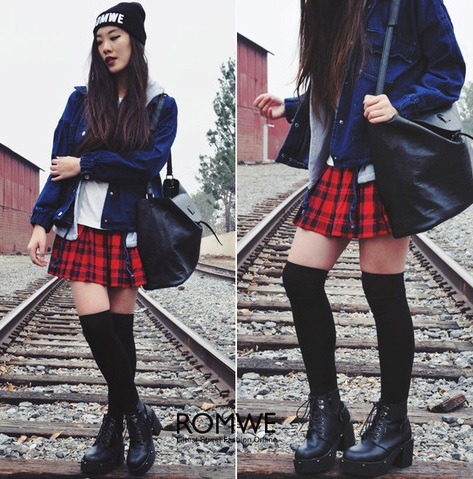This image is a side-by-side composite featuring a young girl modeling an outfit on railway tracks. In the left photograph, she stands on a railroad track, wearing a black toque with white text that reads "ROMWE". Her long, brown hair falls past her shoulders, partially covering her chest. She dons a blue denim jacket over a white shirt, paired with a red and black tartan skirt, which is short enough to reveal her black knee-high socks and dark black ankle boots. A large black purse hangs from her shoulder. The background features an industrial setting with a warehouse to her left and partial view of a tree to her right.

The right photograph provides a closer view of the same girl, from her shoulders down to her feet, giving a clearer look at her black purse, detailed outfit, and boots. The same railway track setting is visible, with the ground covered in rocks. In the background, there's what appears to be either a red barn or a red train station. The company's name "ROMWE" is written in black letters across the bottom of both images, with additional text underneath that is too small to read. This composite image serves as a promotional ad for the clothing and accessories from ROMWE.